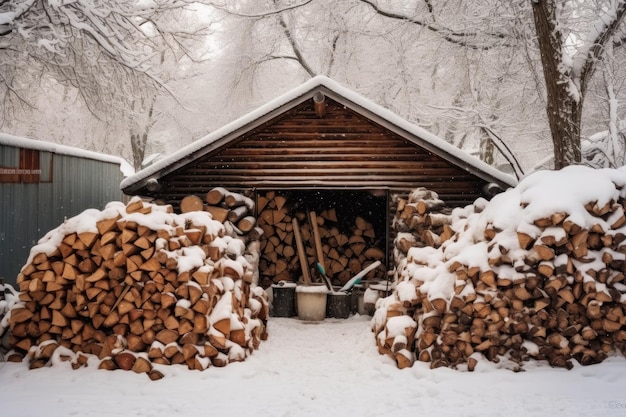The photograph depicts a quaint log cabin shed, centrally framed in a snowy landscape. Constructed from dark brown horizontal logs, the shed features a gabled roof blanketed in snow. The open doorway reveals an interior stacked from floor to ceiling with neatly arranged firewood. Flanking the entryway are two towering piles of cut wood, their ends facing the viewer, each topped with a layer of undisturbed snow, indicating they haven't been used in a while. Several snow-covered buckets, possibly containing tools like an axe and a chainsaw, are scattered in front of the shed. Surrounding the scene is a pristine snow-covered field, with trees in the background also heavy with snow. To the left of the shed, partially visible, is another smaller blue wooden building, similarly coated in snow. The image is a detailed, realistic portrayal of a serene winter landscape emphasizing the tranquil yet utilitarian setting.